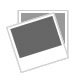This image depicts a yellow soccer jersey hanging on a light brown wooden coat hanger, which is affixed to a metal latch on a white or very light blue wall. The jersey stands out with its shiny yellow fabric and features distinct design elements. There are dark blue stripes running vertically at the top and bottom third of the jersey, while the middle remains a solid yellow. Prominent on the front is the text "Van Mossel Automotive" in blue letters, and directly underneath is a large blue number "2." Further below, in a smaller blue font, the name "Willie Naessens" is displayed. The shoulders of the jersey feature circular blue patterns, and an emblem near the neck area showcases a medieval shield with red, yellow, black, and white colors. The light source seems to come from the upper left, casting a slight shadow at the bottom, enhancing the visibility of the jersey's details and texture.